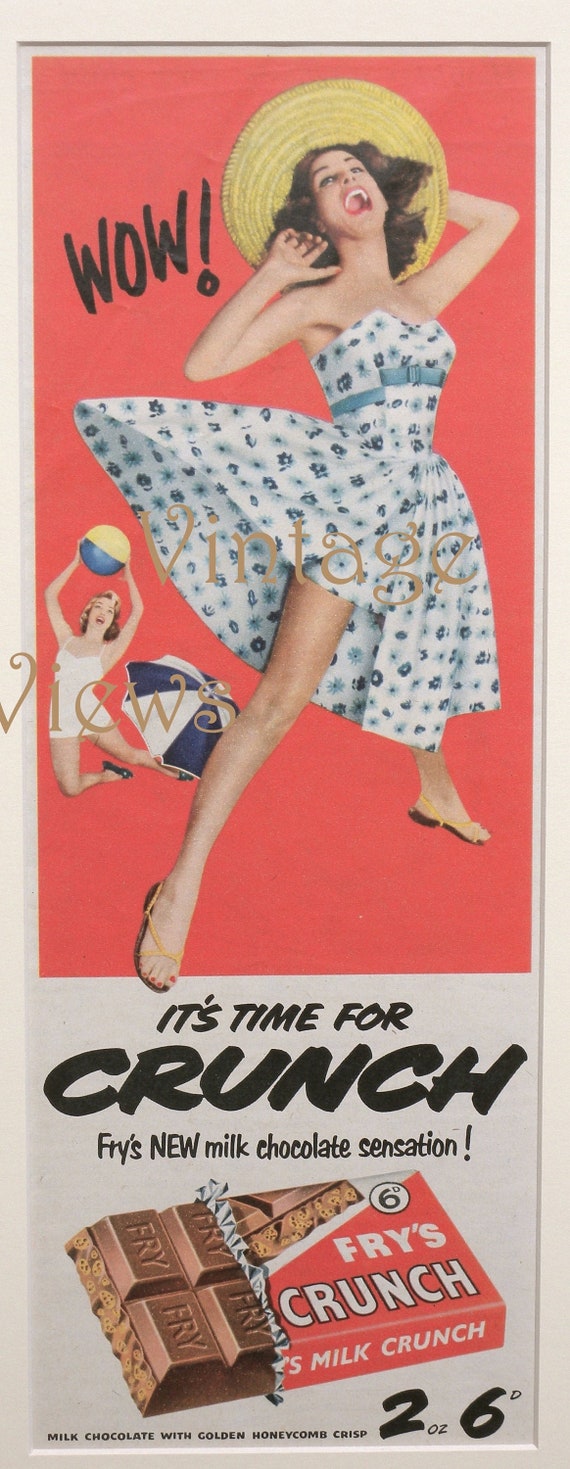This detailed vintage advertisement for Fry's Crunch Milk Chocolate features a vivid and vertically-oriented design. At the top of the image, which occupies approximately three-fifths of the space, there is a striking red background with a woman standing out. She is dressed in a charming white strapless dress adorned with blue floral patterns and accessorized with a white and yellowish beach hat. This woman is captured in a classic pose, with her arms bent behind her head, exuding a timeless, fifties-style glamour. To the left of her head, the exclamation "Wow!" is written in bold black text.

Below her, against a return to a white background, another woman is depicted, this time in a vintage white bathing suit. She is positioned near a blue and white beach umbrella and is holding a beach ball, further enhancing the retro beach theme of the ad. 

Beneath these two women, the background remains white and is framed by a tan border. The text "It's time for Crunch" is prominently displayed in black, leading down to the tagline "Fry's new milk chocolate sensation" in smaller text. An image of the chocolate bar, partially unwrapped, is shown near the text, inviting viewers to indulge. At the very bottom, additional details describe the product as "milk chocolate with golden honeycomb crisp" and offer a promotional deal of "two ounces for $6." The overall high quality of the image and the classic design elements suggest a nostalgic appeal meant to evoke the beloved styles of the late forties and fifties.